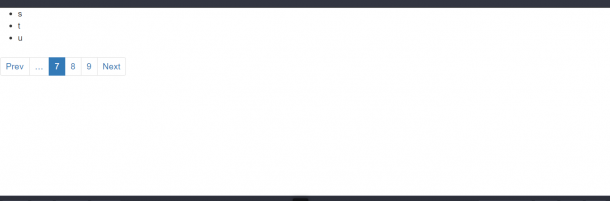The image features a minimalistic page with a white background, leaving much of its surface unoccupied and creating a sparse appearance that makes it difficult to discern whether it is a photograph of a printed piece of paper or a screen capture. 

At the very top of the page, a thick black horizontal bar spans the entire width from left to right. Directly below this bar, in black lowercase lettering with preceding bullet points, are the letters: "•s", "•t", and "•u". 

In contrast to the stark top section, the bottom of the image is more structured, featuring a series of outlined squares in light gray. These squares contain a blue numbering scheme. 

On the left side of this sequence is the word "PREV" in blue. Adjacent to "PREV" are three faint gray dots, leading to a blue square housing the number "7" in white. Following this, a white square displays the number "8" in blue, and next to it, another white square shows the number "9" in blue. Concluding this sequence, the word "NEXT" appears in blue.

Finally, another black horizontal line runs along the bottom of the page, but it is not as wide as the one at the top, creating a visual balance and completing the layout of the image.